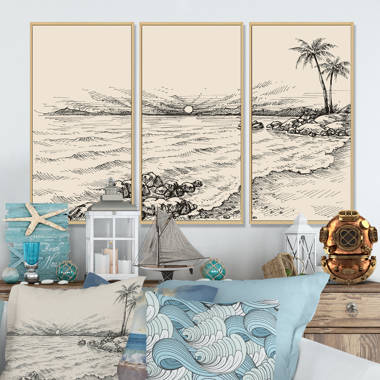This detailed photograph captures a beautifully decorated beach-themed bedroom. Dominating the foreground is a bed adorned with a pillow featuring a vibrant sunset and palm tree design. Adjacent to the bed, there’s an armoire or console table displaying an array of nautical decorations. The first piece is a light blue artwork depicting a beige starfish. Beside it, there is a white lantern housing three candles, followed by a small gray sailboat figure. A round glass object encased in rope sits next to another lantern, which is positioned alongside an antique bronze diving helmet. The wall behind this setup is painted a calming sky blue and features a striking black and white triptych depicting a beach scene with a sunset and two palm trees, rendered in an artistic, pencil-drawn style.